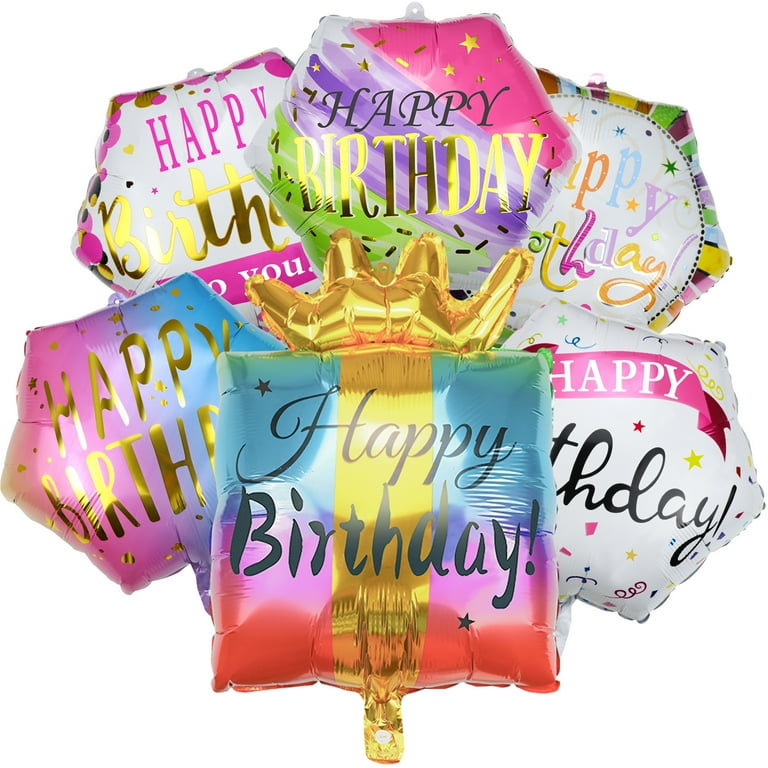This photograph presents a vibrant arrangement of festive Mylar balloons, ideal for a birthday celebration. At the forefront is a square balloon with a striking gold crown, featuring a black "Happy Birthday" text across a gold stripe that runs vertically. The balloon’s design splits into blue on the upper half and pink on the lower half. On either side of this central balloon are two octagonal balloons: the one on the right has a predominantly white background, while the left features a mix of pink and blue hues, each also emblazoned with "Happy Birthday."

Above these, three more hexagonal balloons float. The leftmost balloon sports a white background embellished with pink and gold text, while the rightmost is similarly white but decorated with colors like green and yellow. The central balloon showcases a distinctive rainbow gradient with interspersed stars, bearing a multicolored "Happy Birthday" message. Each balloon's unique design and shape come together to create an eye-catching and celebratory display.